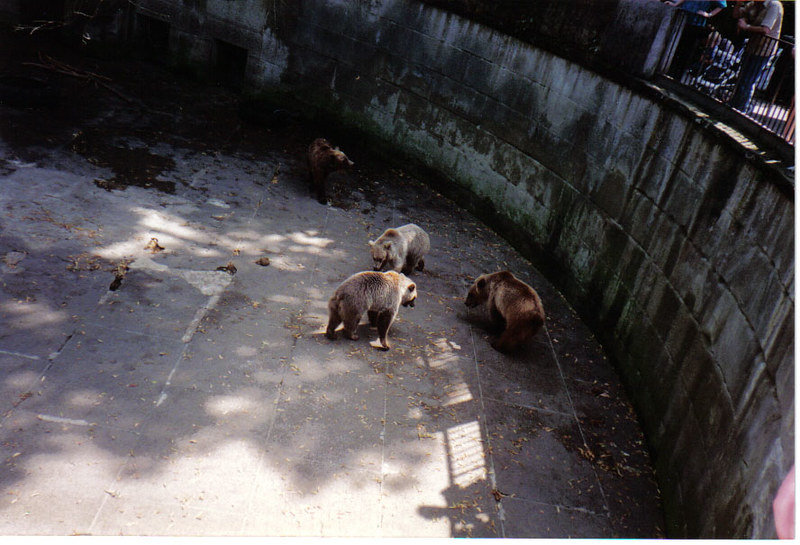This image depicts a zoo enclosure featuring three brown or grizzly bears housed within a large, circular pit. The pit's imposing walls, which are approximately 12 feet tall, are constructed from a gray, moldy, or mildewy stone or cement. The bears are situated near the right edge of the enclosure, clustered together at the center of the image with their snouts down, possibly searching for food among scattered leaves on the otherwise bare, concrete floor. The setting appears bleak and devoid of natural elements like trees, grass, or enrichment items.

Above the pit, a couple of people lean over a railing, observing the bears from a vantage point, creating shadows that cast down into the enclosure. One observer is clearly identifiable in a blue shirt, while the other, partly visible, wears a tan T-shirt. The overall atmosphere of the image emphasizes the stark, uninviting conditions of the enclosure, reminiscent of a cold, gray, and unclean boxing ring.